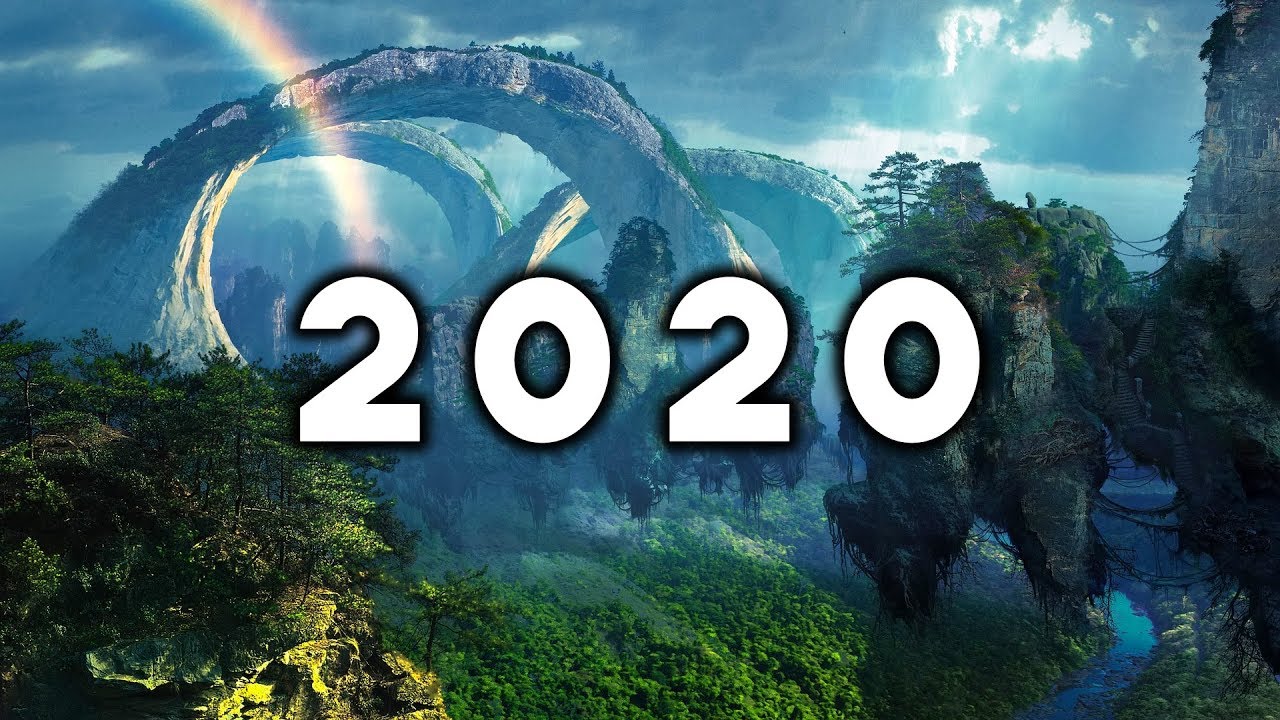This is a digitally generated graphic poster, likely part of a game or comic, showcasing a surreal landscape reminiscent of Pandora from Avatar. Central to the image is the number "2020" written in large, white text with a black outline. The backdrop features a lush, green environment with dark green moss, bushes, and trees. Dominating the background are three large, stone arches, forming interconnected loops that appear to rise out of the ground, resembling tunnels or bridges. The sky above is heavily overcast with dark, gray clouds, though some sunlight peeks through on the right side. A partial rainbow arcs down from the upper left. There's also a small stream visible in the bottom right corner, weaving through the verdant foliage.